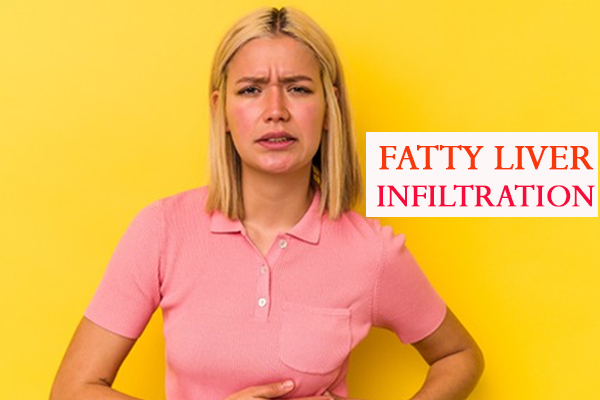The image shows a blonde-haired, white woman standing against a plain yellow background. Her shoulder-length hair is parted down the middle and features darker, black edges at the ends. She is wearing a pink button-up shirt with three clear buttons, two of which are buttoned, and the top one is left open. The shirt has a breast pocket on the left side, visible on the right side of the image.

The woman's face is flushed, with rosy cheeks and expressive features. She has brown eyebrows that are slightly furrowed, brown eyes that are slightly squinting, and a mouth that is pursed open, revealing her top teeth and suggesting a grimace of discomfort or pain. Her ears stick out slightly from beneath her hair.

She is clutching the area around her liver with both hands, with the thumbs of each hand barely visible. Her expression indicates she is experiencing significant discomfort or pain.

On the right side of the image, there is a rectangular white block with text in all red, capital letters that reads "FATTY LIVER INFILTRATION."